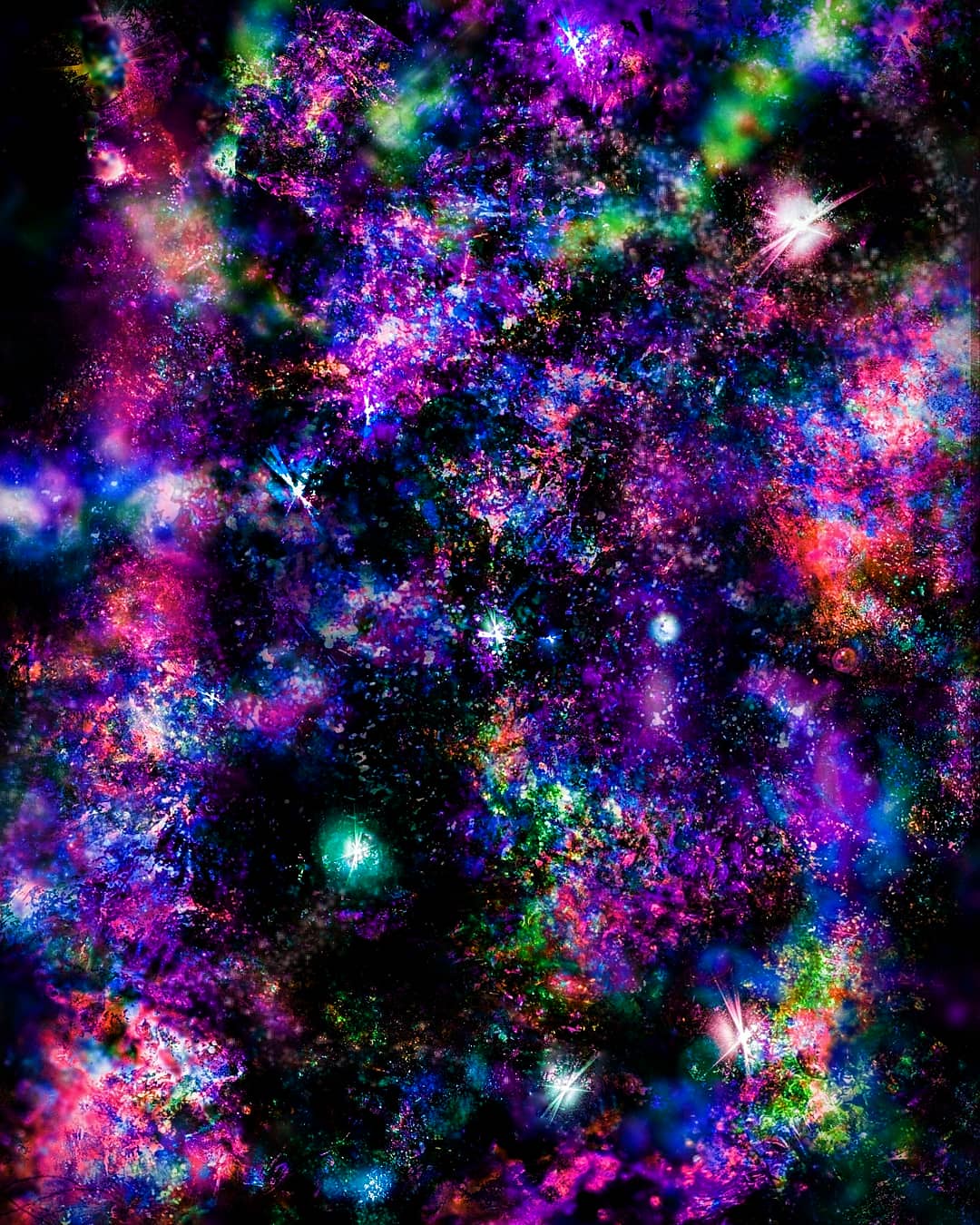The image is an abstract artwork primarily characterized by a black background peppered with bursts of vivid, almost neon colors. The composition is reminiscent of an astronomical scene, with bright flashes and splatters of purple, magenta, green, and blue. These colors blend into cloud-like forms without sharp edges, creating a sense of nebulous expansiveness. Notable elements include a prominent white starburst in the upper-right corner surrounded by splashes of bright green, and a cloudy mixture of white, magenta, indigo, and purple beneath it. In the lower-left section, a turquoise-green circular shape stands out amidst the darkness. Overall, the artwork gives the impression of a vibrant, celestial display set against the profound blackness of space, evoking a sense of otherworldliness and intricate beauty.